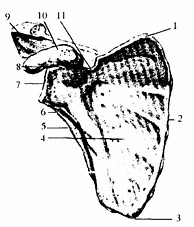This is a highly detailed, hand-drawn, black-and-white scientific diagram possibly depicting an anatomical structure. The illustration is devoid of any identifying labels or legends, making it challenging to ascertain the exact nature of the depicted subject, which could range from an insect's wing to a shoulder blade or even a body part such as a lung or an elephant's ear. The diagram is methodically numbered from 1 to 11, with lines connecting each number to specific parts of the structure. Notably, there is variation in ink density, with the top section being darker compared to the lighter ink used for the majority of the drawing. The image appears more substantial on the right side, while tapering off on the left. Each numbered section lacks descriptive text, leaving the actual identification and function of the parts open to interpretation. The drawing, likely medical or scientific in nature, is sketched on white paper entirely in black ink, giving it a stark, monochromatic appearance.